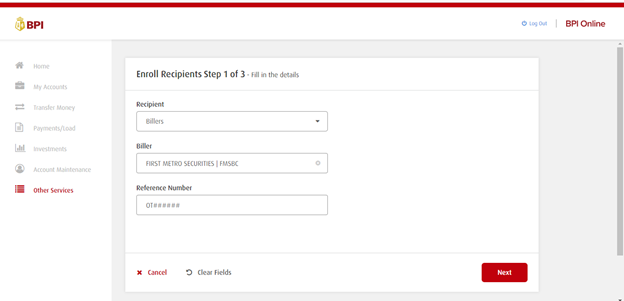In this image, we see the interface of a web page or application page, primarily designed with a white and red color scheme, complemented by gray, black, and red text. At the very top, there is a red bar followed by a white bar featuring the BPI logo on the left side, which is styled in red with a yellow icon adjacent to it. On the far right, there's a blue "Logout" button, and to its right, the text "BPI Online."

On the left-hand side of the page, a menu with options is displayed in gray text, including "Home," "My Accounts," "Transfer Money," "Payments / Load," "Investments," and "Account Maintenance." One option, labeled "Other Services," stands out in red text, indicating it's the currently selected section.

Moving to the main content area on the right of the menu, at the top, there's a heading that reads "Enroll Recipients, Step 1 of 3: Fill in the details." Below this heading, there is a recipient selection box labeled "Billers," which includes a dropdown arrow for more options. Beneath this, within the same section, "First Metro Securities (FMSBC)" is visible as the selected biller. This is followed by a reference number field denoted with "OT#####."

Towards the bottom of the section, there are three buttons: a red "Cancel" button on the left, a gray "Clear Fields" button in the middle, and a red "Next" button on the right.